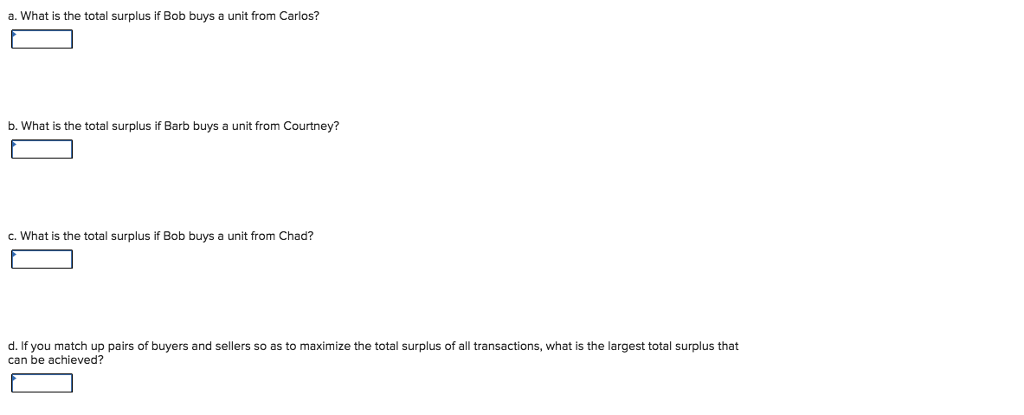**Screenshot of Four Economics Questions on a White Background**

The image is a screenshot featuring four distinct economics questions labelled A, B, C, and D. The background is entirely white, making the screenshot blend seamlessly into a standard page. Each question is followed by a smaller rectangular box outlined in dark blue, with a small blue dot located at the top left corner of each box.

- **Question A:** "What is the total surplus if Bob buys a unit from Carlos?" Below this question is the aforementioned blue-outlined box.
- **Question B:** "What is the total surplus if Barb buys a unit from Courtney?" Similarly, this question has the same blue-outlined box beneath it.
- **Question C:** "What is the total surplus if Bob buys a unit from Chad?" This question also follows the same format with the blue box.
- **Question D:** "If you match up pairs of buyers and sellers to maximize the total surplus of all transactions, what is the largest total surplus that can be achieved?" The same blue-outlined box is present underneath this question as well. Notably, while the top and side lines of the box are blue, the horizontal bottom line appears to be a dark gray. 

Each of the blue boxes shares identical features: blue outline, small blue dot at the top left corner, and a consistent presentation across all four questions.